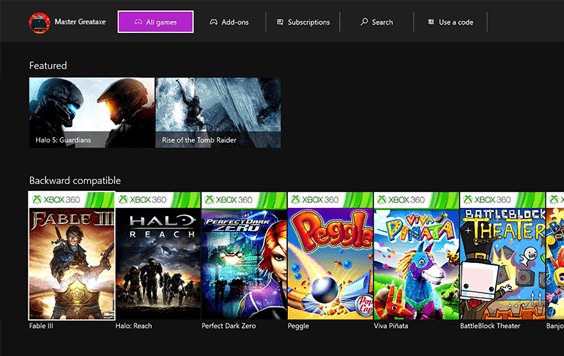The image appears to be a screenshot from the Xbox dashboard, specifically within the games section. At the top left corner, it displays the heading "Master" followed by "Creature." There are multiple navigation tabs aligned horizontally across the screen, starting from the left: "All Games," "Add-ons," "Subscriptions," "Search," and "Use a Code." Below these tabs, there is a section labeled "Featured," showcasing the cover art for two prominent games: "Halo 5: Guardians" and "Rise of the Tomb Raider." Further down, there is another section titled "Backward Compatible," featuring games like "Halo" and "Peggle." The dashboard is designed to help users easily navigate through different game categories and offerings.